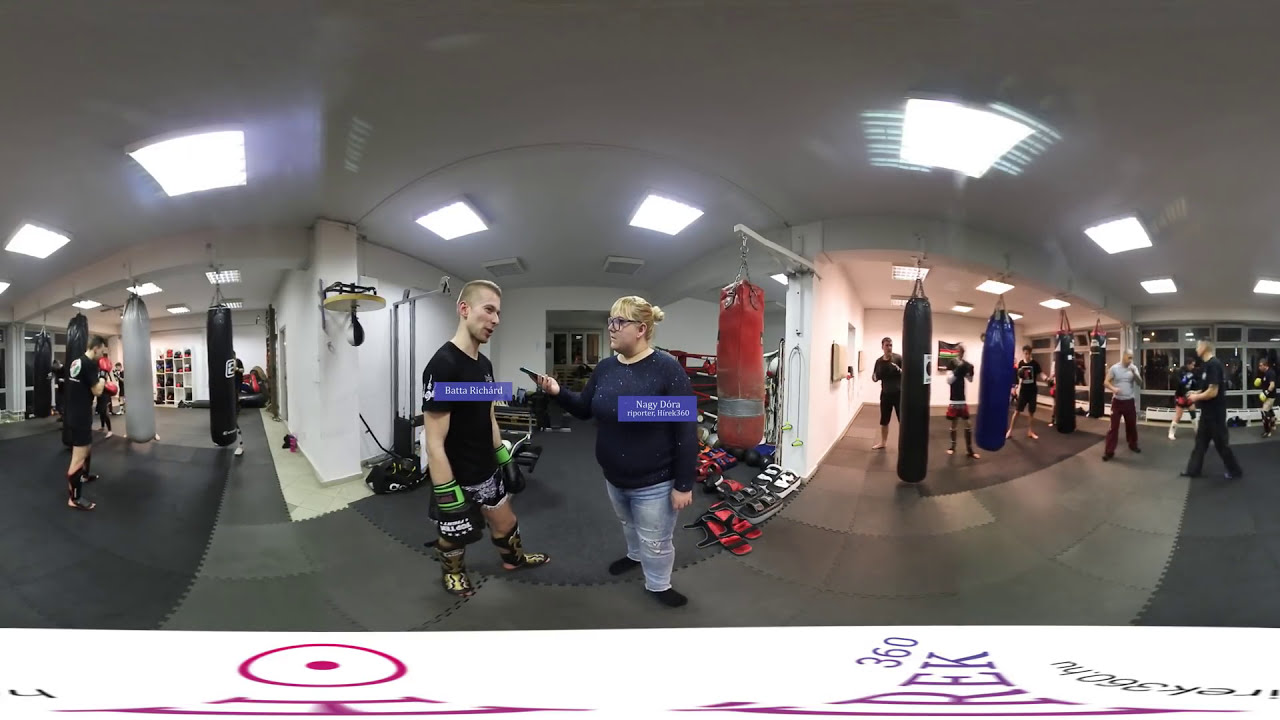This is a detailed panoramic photograph of a bustling boxing gym divided into three distinct spaces by walls. In the first room on the left, there are four punching bags hanging from the ceiling, where a man dressed in all black with red gloves is seen from the back. Moving to the central area, a man with light-colored hair dressed in a black shirt, black shorts, and black gloves with green trim is seen talking to a blonde woman wearing glasses, a long black shirt, blue jeans, and black shoes. They're both surrounded by gym equipment, and a punching bag hovers in the background.

The man and woman appear to be engaged in an interview, with a microphone being held up by the woman, possibly identifying him as the gym owner or a professional trainer. Over their shirts, there are captions, though slightly blurry, seemingly identifying the individuals as Bata Richard and Nagy Dora, suggesting they are not native English speakers.

In the third room on the right, there are four more punching bags where several people engage in their training routine. The gym is packed with numerous individuals kickboxing and boxing, creating a lively and energetic environment. The open space is filled with a variety of equipment, and despite the intensity of the activities, everyone seems to be dedicatedly working out, with signs of sweat and exertion evident.